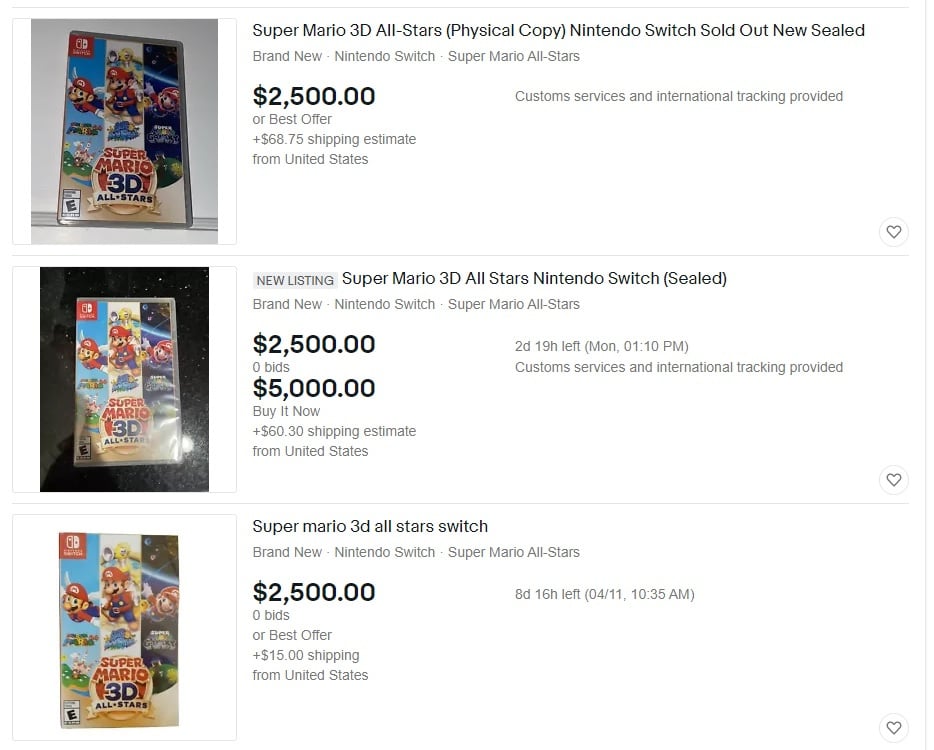**Detailed Description:**

The image is a composite screenshot from a website, divided into three distinct panels, each showcasing a listing for the video game "Super Mario 3D All-Stars" for the Nintendo Switch.

**First Panel:**
The first panel features a listing with an emphasis on a physical copy of "Super Mario 3D All-Stars." The game is rated E for Everyone. The description highlights that the item is new, sealed, and sold out. The price for this brand-new Nintendo Switch game is $2,500, with an additional estimated shipping cost of $6,875. The listing guarantees customs service and international tracking.

**Second Panel:**
The second panel showcases another listing for "Super Mario 3D All-Stars" on a black background. This new listing also offers the game sealed for $2,500. There are currently zero bids, but there is a "Buy It Now" option priced at $5,000. Estimated shipping is $60.30 from the United States. The auction has 2 days and 19 hours remaining, closing on Monday at 1:10 PM. This listing, like the first, provides customs services and international tracking.

**Third Panel:**
The final panel presents yet another listing for "Super Mario 3D All-Stars" on the Nintendo Switch. This brand-new, sealed game is listed at $2,500, with zero bids or best offer options available. Shipping is estimated to cost $15 from the United States. This auction has 8 days and 16 hours remaining, ending on April 11 at 10:35 AM.

Each listing underscores the high demand and value attributed to the game, along with various bidding and shipping options.